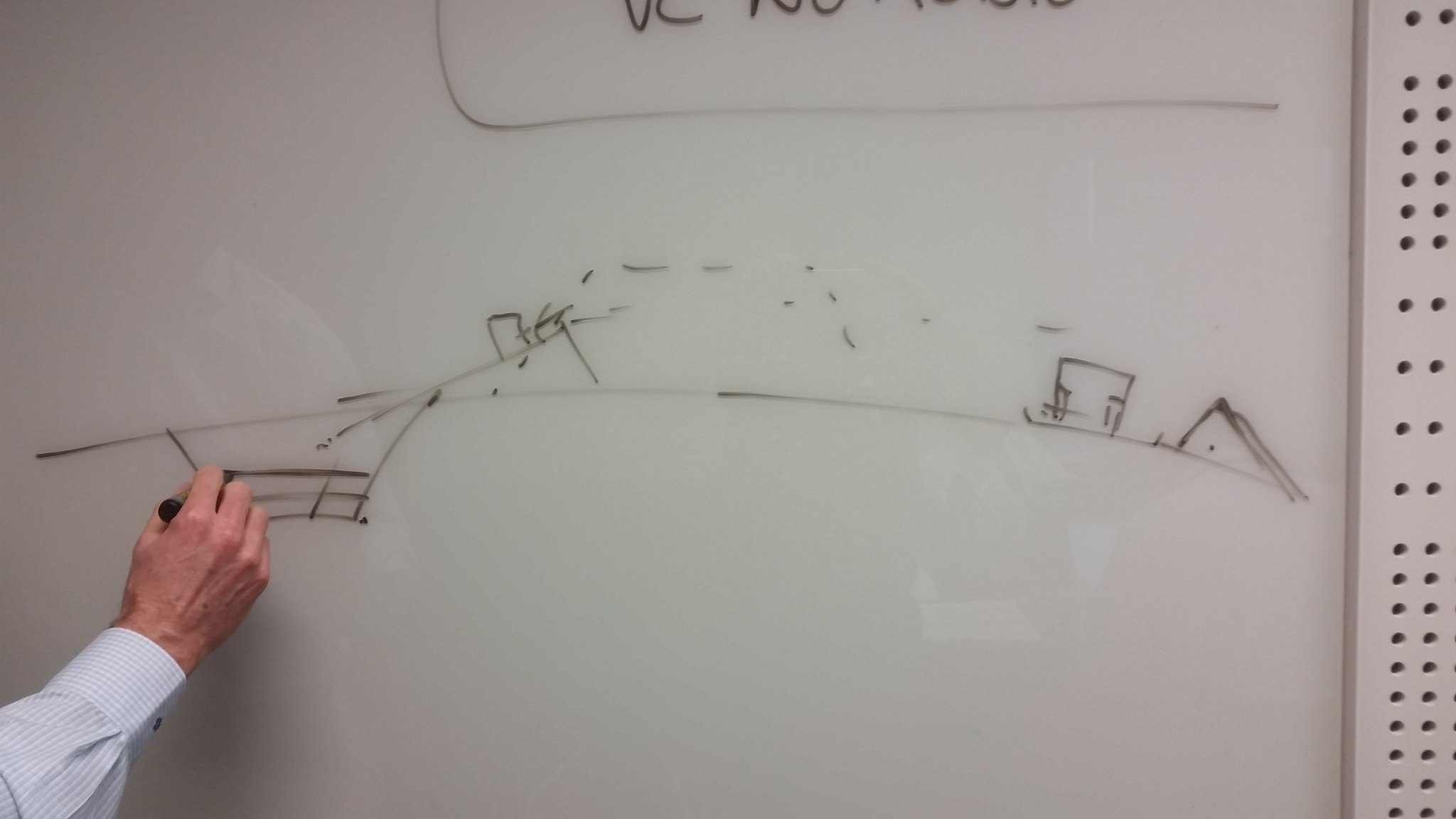In the image, a person is writing on a large dry erase board that nearly fills the entire frame. The whiteboard extends from the top to the bottom and runs almost the whole way across, stopping about an inch from the right edge. Adjacent to the whiteboard on the right side is a white frame or sideboard with a set of holes arranged vertically. Starting from the top, there are two holes followed by multiple groups of two holes with consistent gaps between them, continuing off the bottom of the screen.

Towards the top of the whiteboard, roughly a third of the way in from the left, there is a downward line that curves to the right approximately two inches in, ending an inch from the board's edge. Inside the curved line, there are partial black markings resembling the bottom parts of the letters 'V' and 'L', along with three indiscernible shapes.

In the bottom left corner of the image, a hand, clad in a white dress shirt, is visible. The wrist, top of the hand, knuckles, and partially bent fingers are prominently shown, with the thumb tucked in. The hand grips a black marker, which is visible just to the left of the first knuckle. The marker is constructing a line that starts from the left, near the center of the board, arches slightly upward, and then slopes down towards the right, almost reaching the edge.

From the area near the hand, another line branches downward at an angle, intersecting at the middle knuckle. Three horizontal lines extend rightward from this point, with the bottom line arching upwards before intersecting with the other two lines and continuing upwards to meet an adjacent line. To the left of this formation, a connecting vertical line joins the trio. At the upper connection point, the line angles upward to the right before descending back to the primary horizontal line.

Atop this structure, a small rectangle sits, and further to the right, there is a drawing resembling a small building with front and back windows. Behind this, a 'V' shape is drawn, evoking the image of a distant mountain.